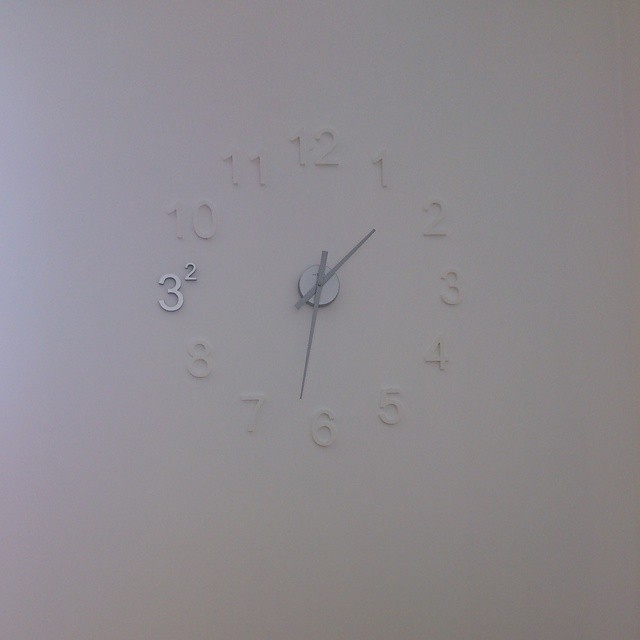This photograph features a largely white wall that, due to poor lighting, appears more gray. On the wall, there is a clock made up of 12 numbers arranged in a circular pattern. At the top of the circle, the number 12 is prominently displayed. The sequence of numbers continues clockwise from 1 through 8, and then unusually includes another 3, which is silver. Positioned slightly above and smaller than this silver 3, there is a smaller number 2. The clockwise sequence resumes with 10 and 11, before returning to 12 at the top. In the center of the clock face, there is a circle containing two silver clock hands.